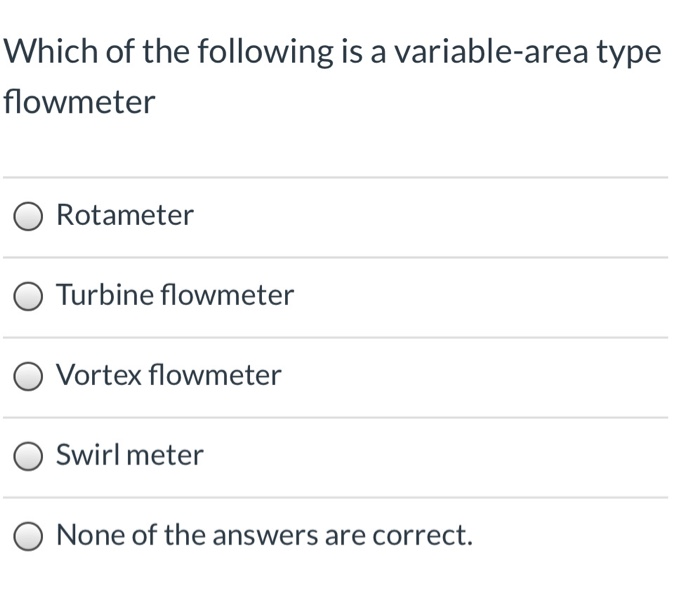A detailed caption for the image could be:

"Screenshot depicting a multiple-choice question with a white background. At the top, the header reads, 'Which of the following is a variable area type flow meter?' Below the question, there are five answer choices, each accompanied by a light gray circular radio button to indicate selection options. Each choice is separated by a thin gray border, resembling a form or table layout commonly found in spreadsheets or online surveys. The choices listed are: 'Rotameter,' 'Turbine Flow Meter,' 'Vortex Flow Meter,' 'Swirl Meter,' and 'None of the answers are correct.' All options maintain a uniform appearance, with gray-filled circular buttons placed to the left of each option for selection purposes."